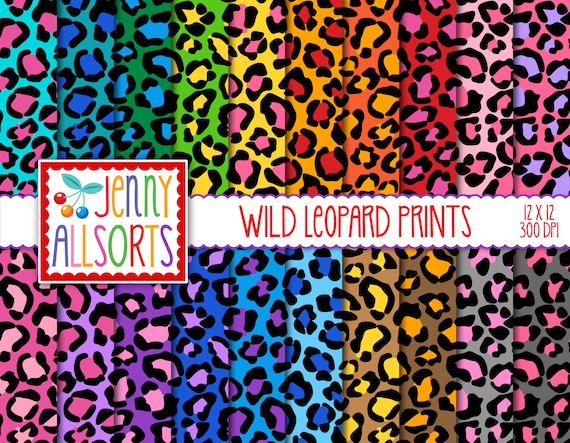The image depicts a collection of vibrant leopard print patterns, each presented in different bold and vivid color combinations including hot pink, teal, aqua, blue, yellow, green, red, and more. There are 20 variations in total, with 10 on the top and 10 on the bottom, layered systematically to showcase the diversity. Each leopard print features a consistent design, where color combinations alternate between the background and the spots, which sometimes include a black outline for added definition. Centrally placed through the image is a white ribbon bearing the text "Wild Leopard Prints, 12 by 12, 300 dpi" and a rectangle with a red border that reads "Jenny Allsorts." This detailed display appears to be aimed at digital scrapbooking enthusiasts, emphasizing the versatility and boldness of the design.